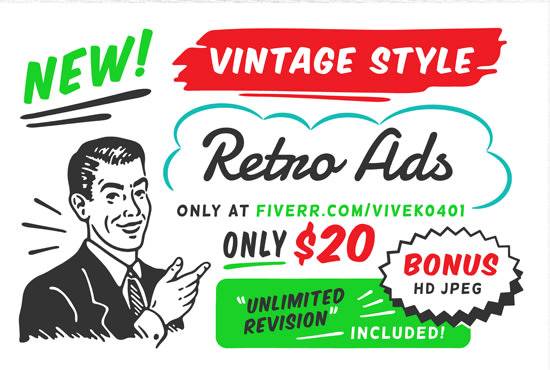This advertisement showcases a vintage-style design that exudes the charm of early 20th-century ads, particularly those from the 1930s, 1940s, and 1950s. At the very top of the ad, the word "NEW!" is prominently displayed in green text, underlined by two black lines, delivering a bold announcement. To the right, in a striking red background with white text, it reads "VINTAGE STYLE."

Centrally placed in varied retro fonts and colors is the enticing offer: "RETRO ADS, Only at Fiverr.com/vivec0401." This is followed by the details, "Only $20, Unlimited Revisions Included, Bonus HD JPEG," inviting potential customers with promises of quality and satisfaction.

In the lower left-hand corner, there is a detailed, hand-drawn picture of a gentleman wearing a black jacket, striped tie, and white button-up shirt. His vintage hairstyle and the retro art style, reminiscent of the 1940s and 1950s, reinforce the nostalgic theme. The gentleman is depicted pointing at the ad, compelling viewers to pay attention to the irresistible offer.

This advertisement is a perfect blend of nostalgic aesthetics and modern-day convenience, bringing forth a meticulously crafted retro design that promises value and authenticity.